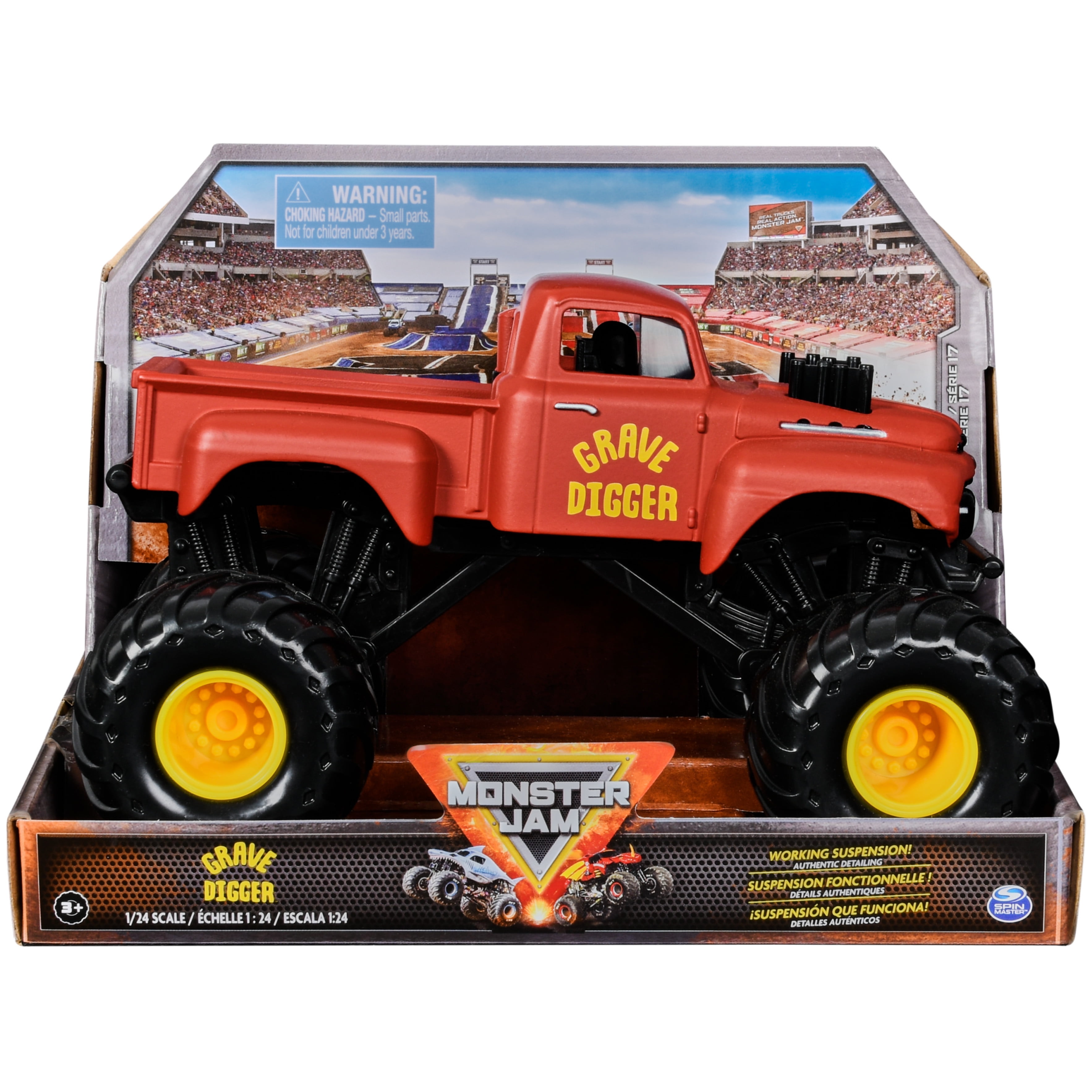The image depicts a red "Grave Digger" monster truck toy encased in its original packaging. This toy, part of the Monster Jam series, showcases the truck with massive black wheels equipped with yellow hubcaps. The truck, emblematic of the Monster Jam arena, features "Grave Digger" written in yellow font on the side door. The packaging, a cardboard box with a stadium backdrop, prominently displays various details. At the bottom inside an upside-down triangle, the Monster Jam logo is visible. The box also states "Grave Digger" and provides essential information, such as the toy’s 1:24 scale size, the working suspension feature, and a warning about it being a choking hazard for children under three years of age. Additionally, the warning is repeated in two other languages.